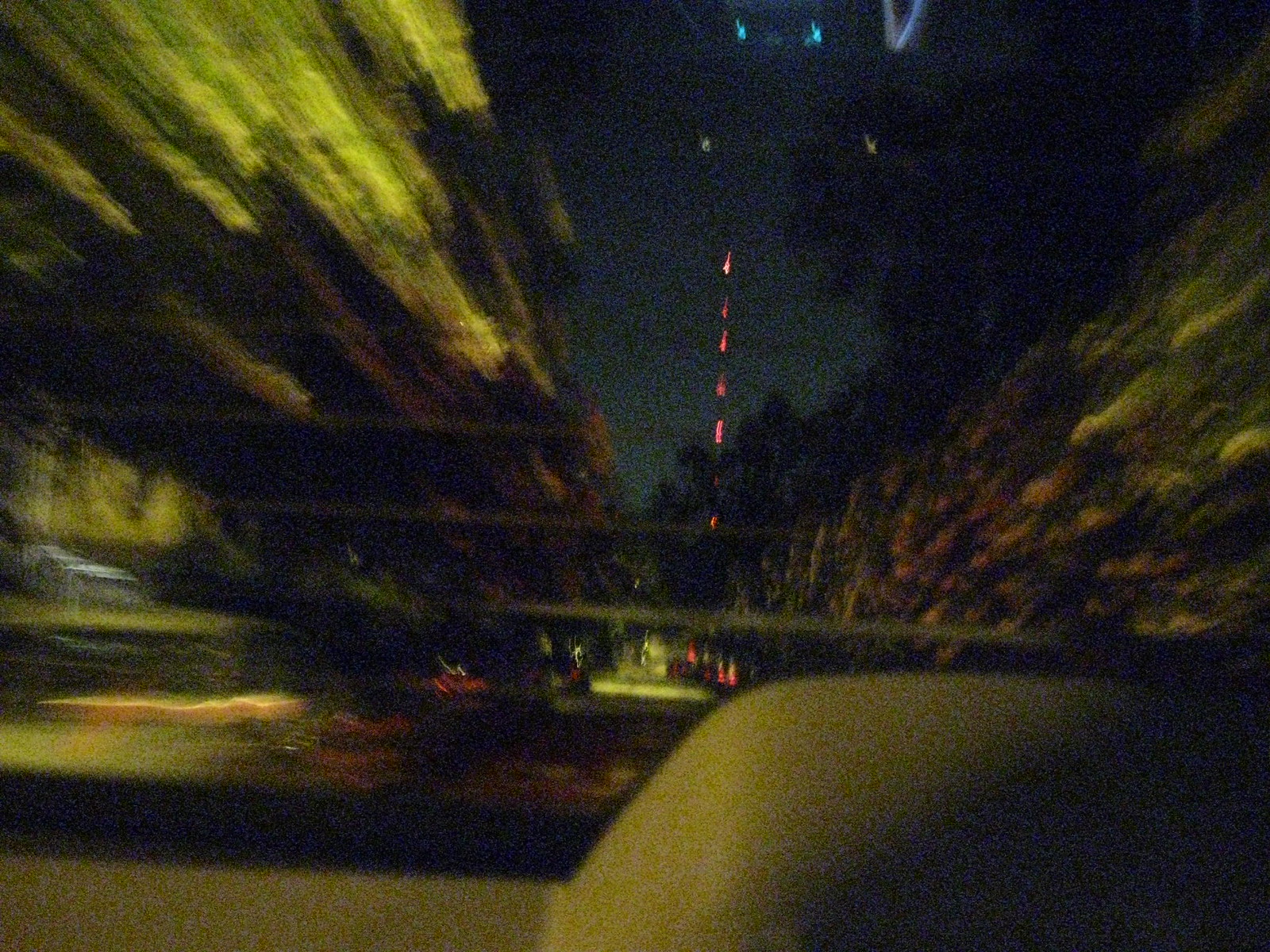The photograph captures a scene from the backseat of a car, framed through the rear window with its horizontal defroster lines clearly visible. The lower part of the image shows the upper edge of the car seat, offering a sense of the car's interior. Outside, the blurred motion of the surroundings suggests that the car is in motion. On both the left and right sides of the window, large green bushes or trees fill the view; the foliage on the left side is a lighter shade of green, while the vegetation on the right is a darker hue. In the distance, a dirt road stretches out, flanked by an orderly array of orange traffic cones guiding the path. Above, the sky looms ominously dark, almost black, adding a moody atmosphere to the scene. Red lights or reflections streak down the center, their origin ambiguous—whether within the sky or as a result of a reflection remains unclear.